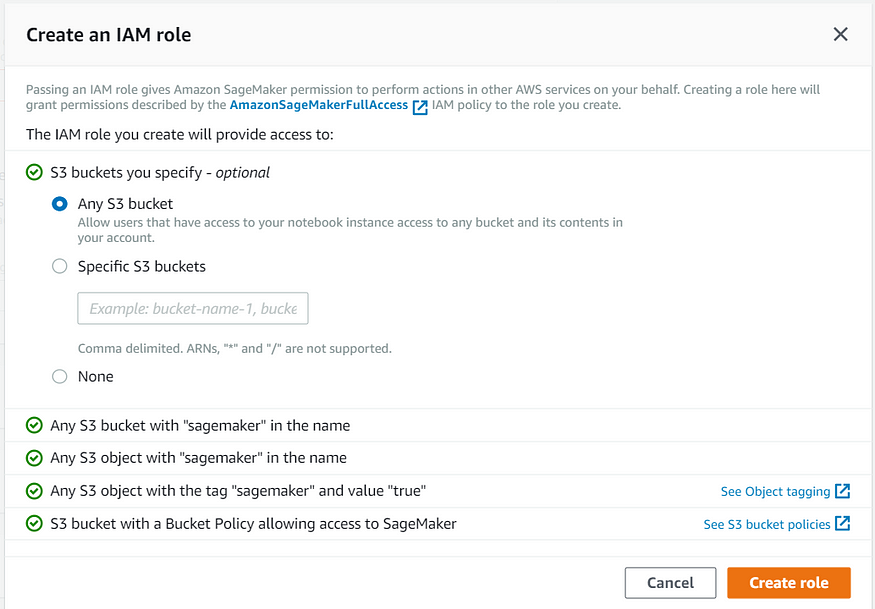This screenshot displays the settings tab of an application focused on creating an IAM role. At the top, "Create an IAM Role" appears in dark bold font, accompanied by an 'X' on the right to exit the tab. Just below, a smaller gray text explains that passing an IAM role provides Amazon SageMaker the permissions needed to perform actions in other AWS services on your behalf, followed by a longer disclaimer.

Further down, "The IAM role you will create will provide access to" is written in bold, small black font, followed by three options: "Any S3 bucket" (selected with a checkmark), "Specify S3 buckets," and "None." The selection list for "S3 buckets that you specify" appears to the left, with four more categories in the pop-up, all of which are also checked.

At the bottom of the tab, on the left side, you find the "Create" option, whereas on the far bottom right, there is an orange "Create role" button. Just to its left, a "Cancel" button is also available.